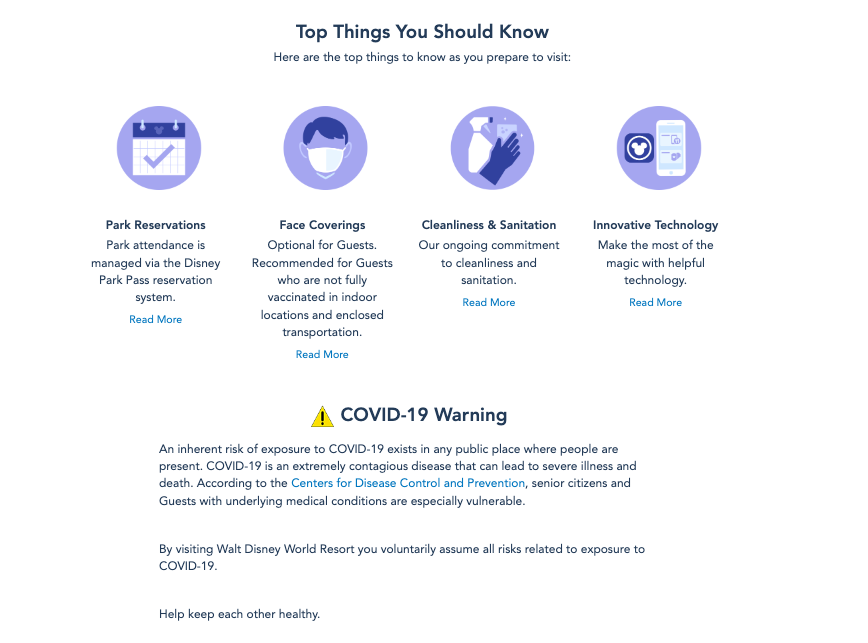**Top 10 Things You Should Know for Your Disney Visit**

In this informative guide, we highlight key points to help you prepare for your Disney visit. The image is headlined with four prominently placed blue circles, each containing an illustrated icon that corresponds with essential information.

1. **Park Reservations**: The first circle emphasizes the importance of making park reservations. Attendance is managed through the Disney Park Pass reservation system to ensure a smooth experience for all guests.

2. **Face Coverings**: The second circle details the current policy on face coverings. While optional for guests, face coverings are recommended for those who are not fully vaccinated, particularly in outdoor locations and indoor transportation.

3. **Cleanliness and Sanitation**: The third circle highlights Disney's ongoing commitment to maintaining cleanliness and sanitation throughout the park to ensure the safety and well-being of all guests.

4. **Innovative Technology**: The fourth circle encourages guests to utilize Disney's innovative technology to enhance their visit, offering helpful tools to make the most of the magic.

Each of these points includes a "Read More" link in blue for further details.

Below this informative section, a bold, centered heading reads: **COVID-19 Warning**. A critical paragraph follows, outlining the inherent risks associated with COVID-19:

"Exposure to COVID-19 is a risk in any public place where people are present.